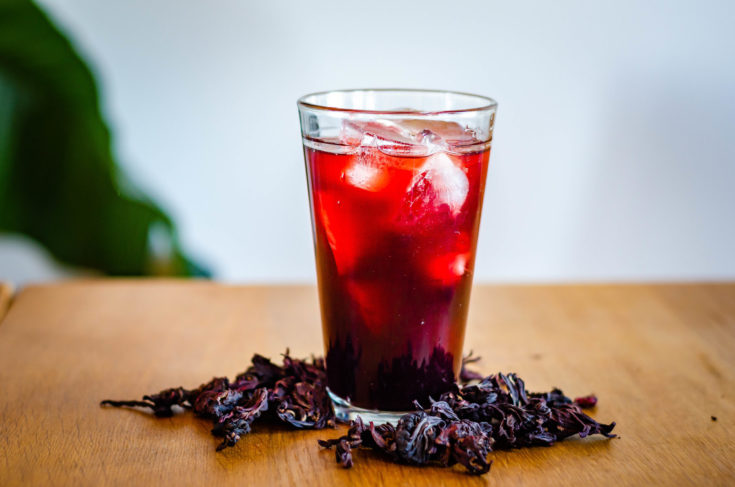The horizontally aligned close-up image features a clear, tall pint glass filled with a reddish liquid, almost to the brim, resting on a medium-brown wooden table with subtle thin grain patterns. The drink inside the glass has a gradient, appearing darker red, almost purple at the bottom, and becoming lighter and more transparent towards the top. Several large, see-through ice cubes float within the liquid. Surrounding the base of the glass are purplish-black, raisin-like herbs or spices. The background of the image is blurry, displaying a light gray wall with a large green leaf descending from the upper left-hand corner.